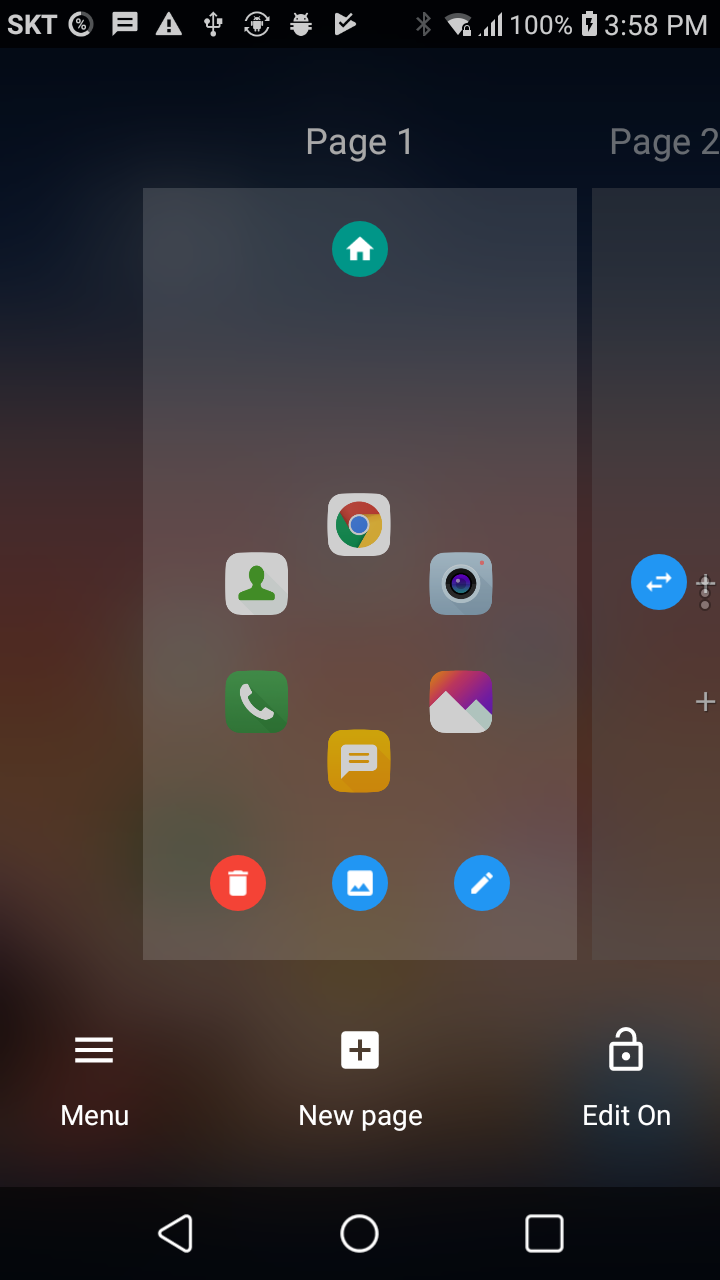Screenshot of an Android Phone Home Screen Taken at 3:58 PM

At the very top right corner, the screenshot displays the current time, 3:58 PM. To the left of the time is a fully charged battery icon with a lightning symbol inside it, indicating that the phone is currently plugged in. Adjacent to the battery icon, the phone signal strength is at full bars, while the WiFi signal strength is one bar short of full. The Bluetooth icon next to the WiFi signal is grayed out, showing it's turned off.

On the left side of the status bar, the letters "SKT" identify the network provider. To the right of these letters are several smaller icons: the first is a circle, followed by a message notification icon, a triangle with an exclamation point, a USB connection symbol, and finally, two Android system icons.

In the main part of the image, a square box prominently displays several app icons without labels. Among these, the Google Chrome browser icon, a camera icon, a photo gallery icon, a messaging app icon, a phone dialer icon, and a contacts icon can be identified.

This detailed observation highlights not just the layout but also the functionality statuses of various features on the device's home screen.